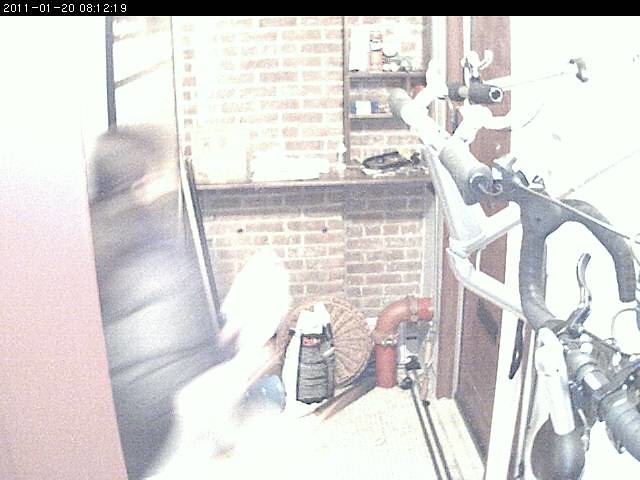A detailed and high-resolution image of a utility room featuring a prominent brick wall and an older chimney positioned centrally. The room details numerous water and drainage pipes entering and exiting the building, complete with various types of valves, including lever valves and ball valves. On the right side, there are multiple spliced lines. The left side of the image captures a blurry figure, possibly an individual in motion either turning or entering the room. The overall setup, including the piping arrangement, placement of valves, and shelving units, hints that the image may have been generated by AI due to certain inconsistencies such as improperly attached pipes, jutting drain pipes that aren't fully connected, and noticeable gaps. There are also strange angles in the piping that a professional plumber would likely avoid. This grainy image emits an uncanny ambiance, suggesting that it may not be a real-world photograph but rather an AI-generated depiction of a utility room.